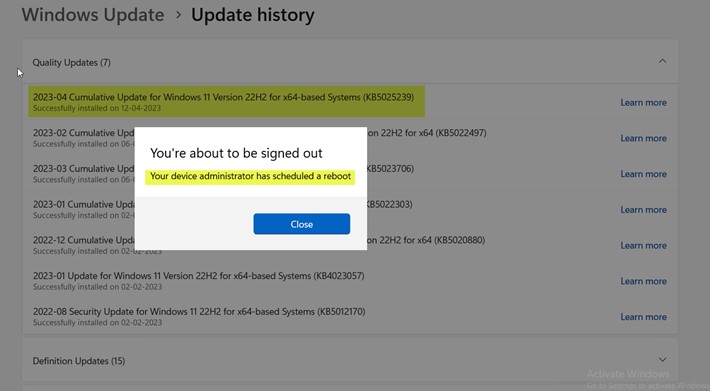Screenshot Description:

The screenshot displays a Windows Update screen with a focus on the Update History page. At the top, there's a title that reads "Windows Update," followed by a direction arrow pointing to "Update History." The main section is divided into two columns: on the left, titled "Quality Updates," and on the right, listing various update events with their respective month, year, and brief descriptions.

The first update event is labeled "Cumulative Update for Windows 11 Version 22H2 for x64-based Systems," complete with an update ID number in parentheses. Each event title is followed by a blue "Learn More" link in the second column. The initial row is highlighted in yellow to draw attention, while the subsequent rows have a plain white background with black text. The entire Windows Update History area is currently grayed out, indicating that it is not interactive at the moment.

Above this section, a white pop-up window emerges, prominently stating, "You're about to be signed out." Below this notification, highlighted in yellow, it mentions, "Your device administrator has scheduled a reboot." At the bottom of the pop-up, there is a blue button with white text labeled "Close."